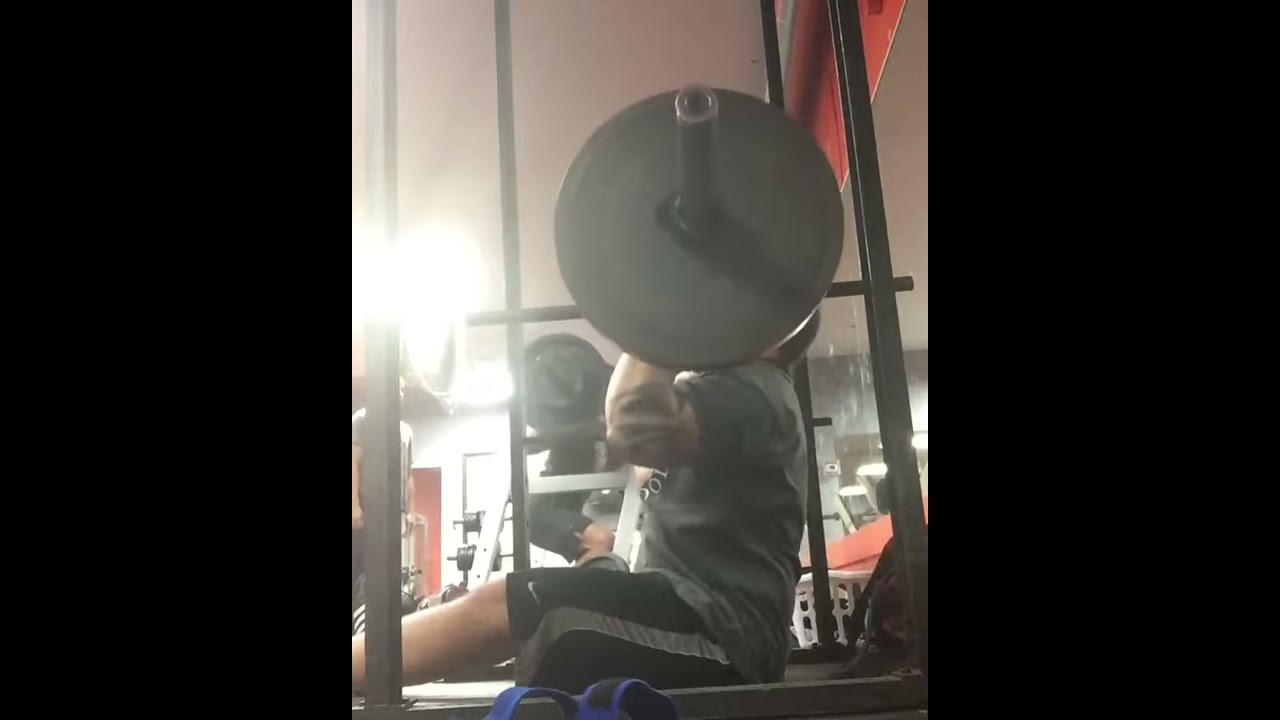In the image, we see a person seated on a weight bench engaged in a shoulder press exercise. The individual's head is obscured by a weight plate, approximately 15 inches in diameter, which is mounted on a weight bar. His short black hair is partially visible at the back. He is wearing a dark gray shirt with indistinct lettering, along with black shorts that feature a Nike logo and a gray stripe running down the side. His left arm and shoulder, exhibiting a tattoo near the elbow, are clearly visible, as are his lower torso, kneecap, calf, and shin.

The setting is an indoor gym, evidenced by various pieces of exercise equipment and weights visible throughout the scene. A mirror is located on the right side of the image, while on the lower left corner, additional weight machines are distinguishable. There is also an overexposed light source on the left edge of the image, causing a noticeable flare. In the background, a white wall with a red door can be seen. Another individual, somewhat blending into the surroundings, stands in the back, wearing a black shirt and gray pants. The image is captured in a portrait vertical orientation, showcasing a varied color palette of black, white, tan, gray, red, orange, and blue.